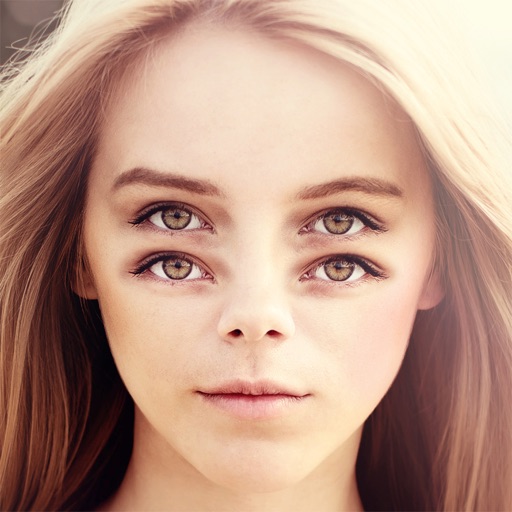This image appears to be a digitally manipulated close-up of a young woman with four eyes, which makes the composition quite unsettling. Her face dominates the frame, leaving no background visible, suggesting a professional and highly controlled photographic setting. 

The woman, who appears to be Caucasian, has blonde hair that is especially vibrant at the top right due to the lighting, although it transitions to a darker blonde shade towards the inside. Below her dark blonde eyebrows, she has two sets of hazel eyes positioned on each side, one directly above the other. The manipulation is evident in the slightly unnatural shadows and depth around the extra eyes, which seem to have been copy-pasted in a crude manner. 

Her small nose is positioned centrally below the two sets of eyes, and her hair cascades down in front of the tops of her ears. Her lips are pink but appear dry. The image's color palette includes shades of blonde, hazel, brown, tan, black, olive, and pink, contributing to the overall distorted, yet striking visual effect.